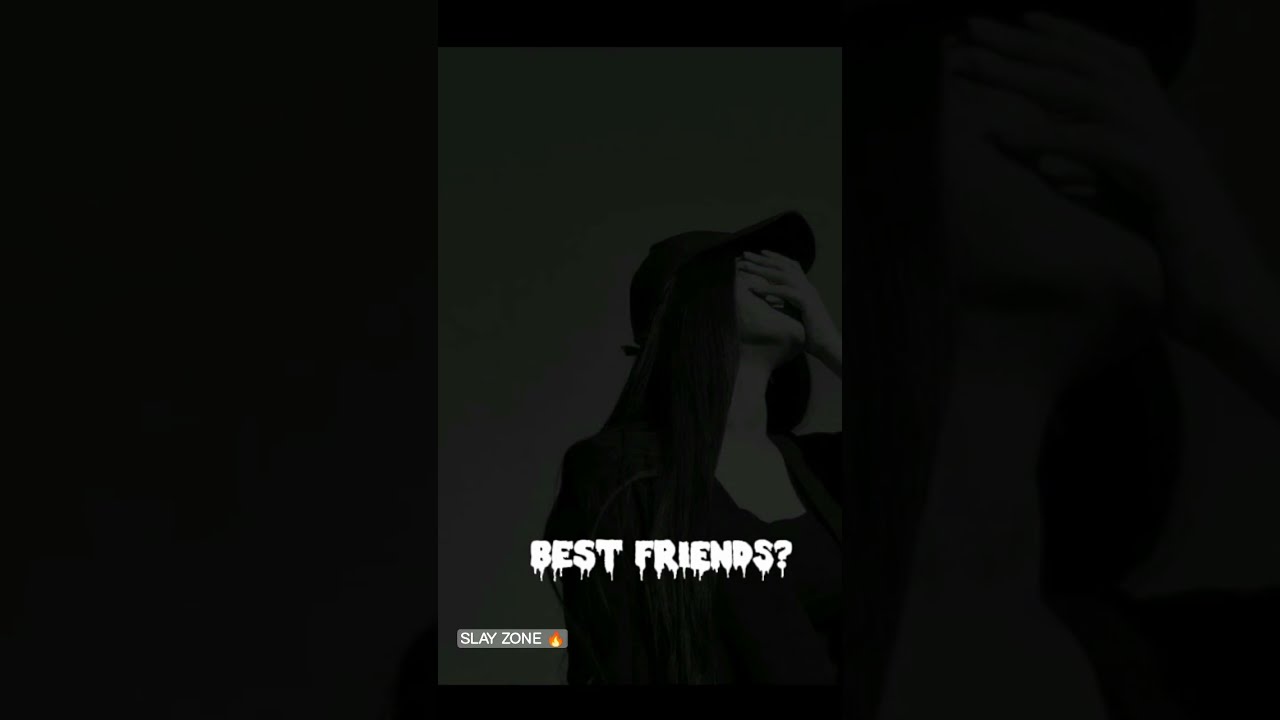The rectangular image, approximately twice as wide as it is tall, is divided into three horizontal sections, with the leftmost and rightmost sections appearing as plain black fields void of any features. Dominating the center section is a heavily darkened photograph of a woman, possibly wearing long dark hair and a black baseball cap, or some type of head covering. The obscured face of the woman is partly hidden by her hand, leaning slightly back, and she is dressed in what appears to be a black top. The entire photo is low in exposure, making details difficult to discern. Across her chest in the center, white text with a dripping, almost blood-like appearance reads "Best friends?" Toward the lower left corner, a gray box with white text states "Slay zone" followed by a fire emoji.